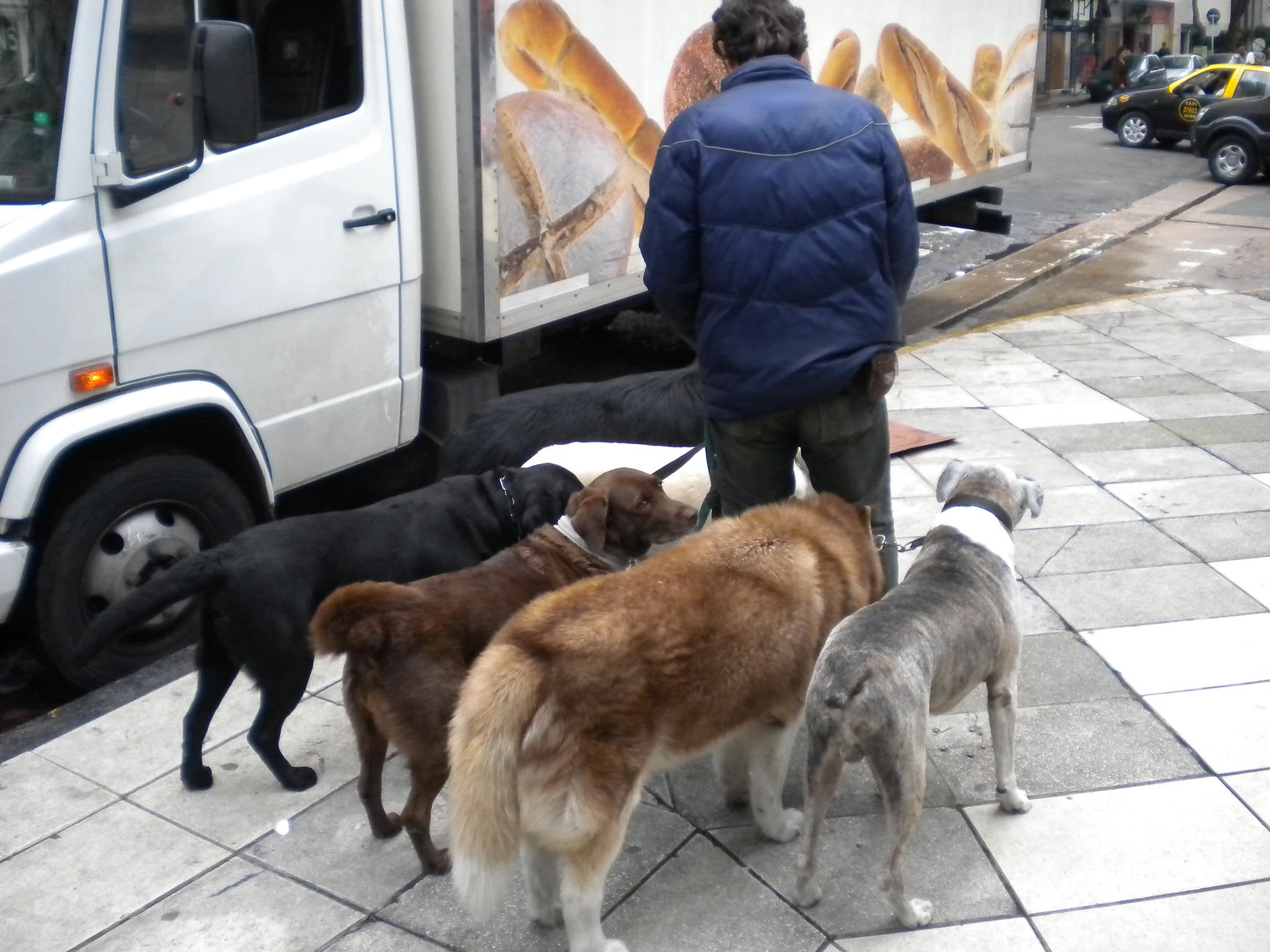The photo captures a scene on a European city street dominated by a man walking six dogs on leashes. The man, dressed in a blue puffer jacket and dark jeans, stands in the center of the image, with his back to the camera. He appears to be looking down at one of the dogs, perhaps giving it some attention. His short, dark hair curls slightly around his ears. The sidewalk beneath them is made of square paving slabs in shades of grey, white, and beige, arranged in a patterned mosaic.

Behind the man and his dogs, a white delivery van with images of various loaves of bread covers much of the left side and top middle of the photo, indicating it might be delivering to a nearby supermarket. The street scene extends to the top right corner of the image, where you can see a yellow and black taxi cab, other parked cars, and a few pedestrians, all partially obscured by the van and buildings.

The six dogs are of different breeds and colors, all patiently standing on the sidewalk. To the lower right is a grey dog with short hair and a white ruff. Next to it is a fluffy brown and gold dog, possibly a husky. A medium brown dog, likely a Labrador retriever, looks over the back of the husky. There is also a dark-furred dog, potentially a Lab mix, with its head tucked down and tail extended horizontally. Two more dogs stand to the left of the man; one is white and the other is black, although their heads are cut off by the man's body and the other dogs. The man holds all the leashes in front of him, maintaining control over the diverse pack.